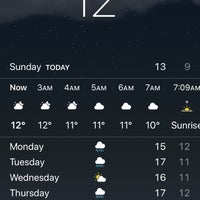This image is a cropped screenshot from a smartphone, focused on a weather forecast app. The screen's top portion, showing the time "12" in white, is partially cut off due to zooming. The black background contrasts with the white numerals, making the cut-off digits noticeable. Below the time, the screen displays the date "Sunday, today," with a high of "13" and a small "9" next to it, most likely representing the low. 

The forecast indicates that as of now, it is partly cloudy with a temperature of 12 degrees. The hourly forecast shows a steady temperature decline: 
- 3 AM: 12 degrees, partly cloudy
- 4 AM: 12 degrees, partly cloudy
- 5 AM: 11 degrees, partly cloudy
- 6 AM: 11 degrees, fully cloudy
- 7 AM: 10 degrees, fully cloudy

A note next to "7:09 AM" states that sunrise occurs at this time. 

On the left side of the screen, upcoming days are listed:
- Monday
- Tuesday
- Wednesday
- Thursday

Each day includes small cloud icons and temperature highs (ranging from 15 to 17 degrees) in white and lows (11 or 12 degrees) in gray.